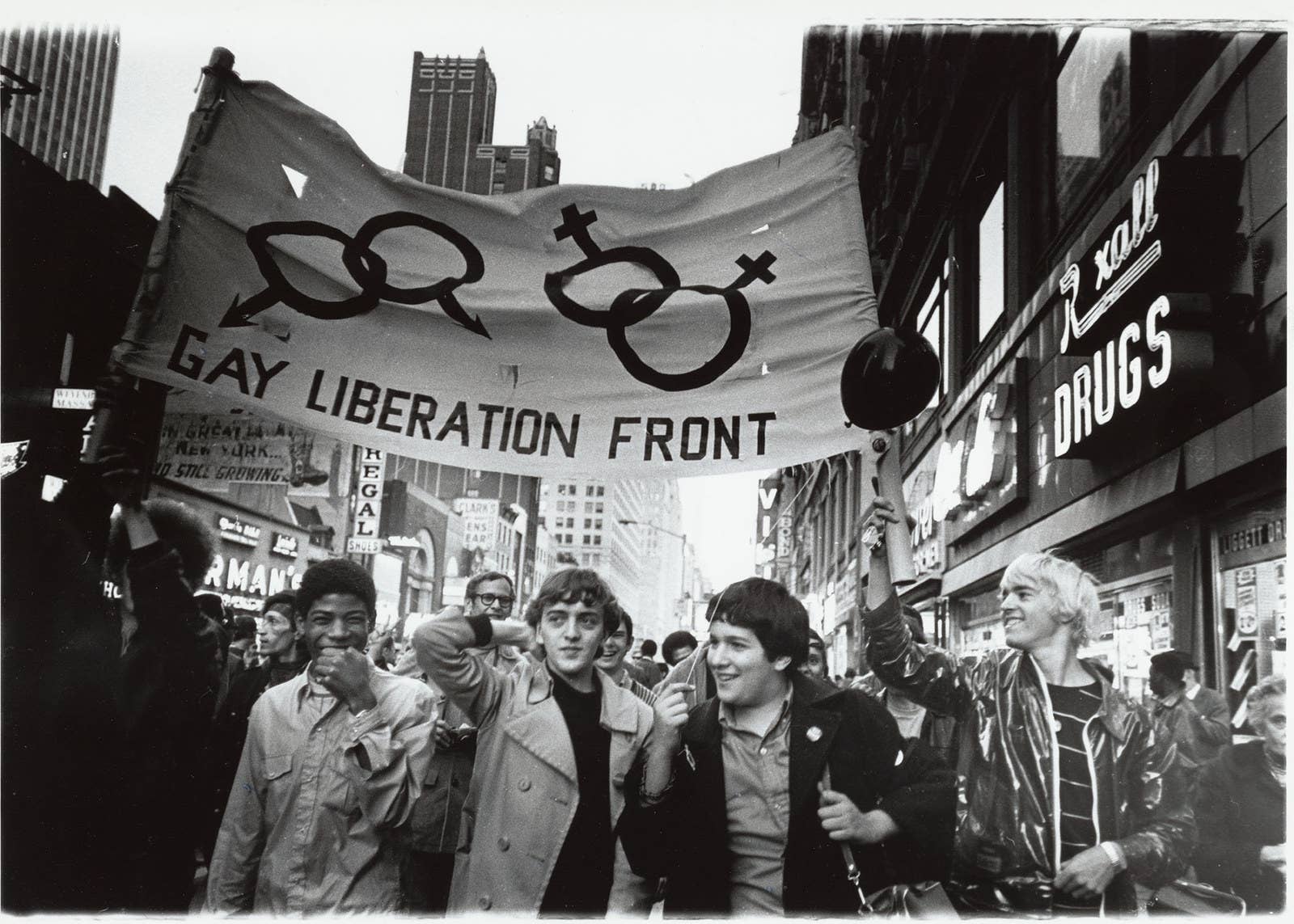This black-and-white photograph captures a vibrant Gay Liberation Front parade in what appears to be a major inner city, likely New York City, given the towering buildings and well-known establishments like Rexall Drugs and the Regal Theater visible in the background. The parade features a diverse group of mostly young men, of mixed races, marching proudly. At the forefront, three smiling young men carry a prominent white banner with the text "Gay Liberation Front" and interlinked gender symbols for males and females. On the right side of the banner, a blonde man, dressed in a jacket, holds one of the supports, embodying the exuberant spirit of the event. The scene is bustling, with bystanders visible on the sidewalk, including an older woman who appears slightly unsettled. The participants, clad in long sleeves, exude joy and camaraderie as they walk through the city streets under the chilly weather, making a powerful statement for gay rights, presumably in the 1980s.